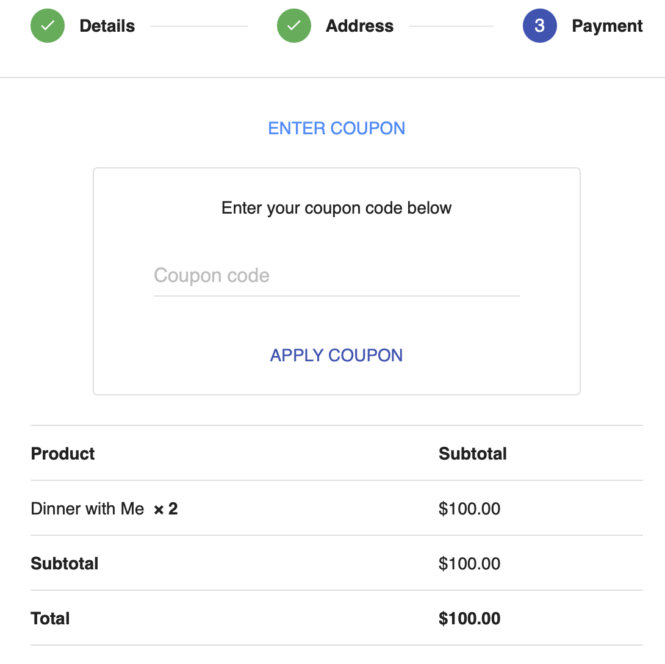The image appears to be a checkout or payment page from a website, characterized by three distinct sections at the top: 

1. A green circle with a checkmark labeled "Details."
2. Another green checkmarked circle labeled "Address."
3. A blue circle with the number three in it labeled "Payment."

Below these sections, in blue text, the option to "Enter Coupon" is presented. 

There is a prominent box instructing users to "Enter your coupon code below." Within this box, a light gray placeholder text "Coupon Code" appears above an underlined field for input. Below this field, in bluish-purple text, users are prompted to "Apply Coupon."

Further down, the page is segmented into columns under the headers "Product" and "Subtotal." Listed under "Product" is an entry for "Dinner with me times two" which totals $100. The subtotal and total are both displayed in bold as $100, indicating no discounts or additional taxes have been applied.

The page appears to be for a nondescript dinner reservation or meal purchase, as no restaurant name or further details are provided. This image highlights an interesting aspect of the checkout process but leaves the context and specifics of the purchase quite ambiguous.